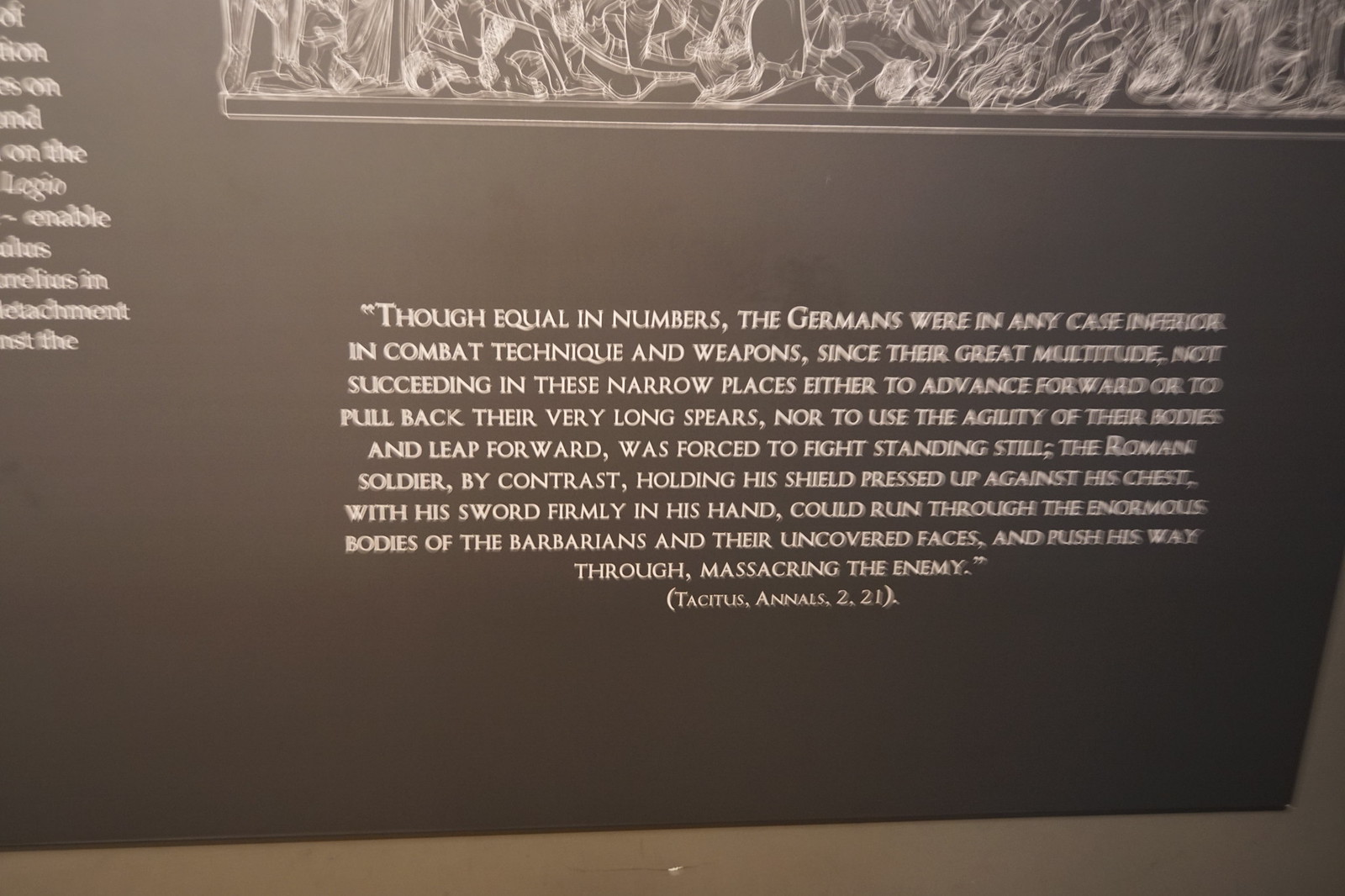The image depicts the bottom portion of an informational sign from a museum, featuring a detailed quote in white, small-cap lettering on a black background. Above the quote, there is a blurred image or drawing, flanked by some indeterminate, partially cut-off text in the upper left. The main content is a historical quote attributed to Tacitus from "Annals 2.2.1." It reads: "Though equal in numbers, the Germans were in any case inferior in combat technique and weapons, since their great multitude, not succeeding in these narrow places either to advance forward or to pull back their very long spears, nor to use the agility of their bodies and leap forward, was forced to fight standing still. The Roman soldier, by contrast, holding his shield pressed up against his chest with his sword firmly in his hand, could run through the enormous bodies of the barbarians and their uncovered faces and push his way through, massacring the enemy." The dark background and the structured format give the quote a solemn and authoritative presence, emphasizing the historical narrative.